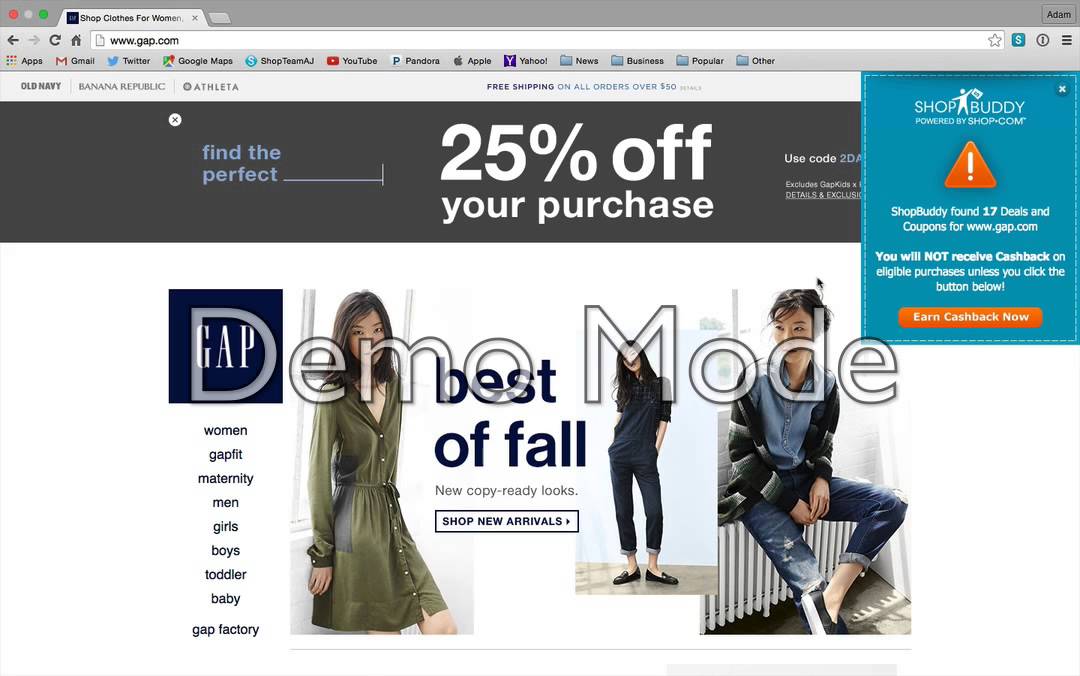This screenshot captures a desktop view of a Mac operating system, indicated by the characteristic traffic light icons in the upper left corner—red, yellow, and green. The browser tab is open to the official website of the clothing retailer GAP, with the URL www.gap.com visible. The tab is titled "Shop for clothes for women," confirming that the page is dedicated to women's apparel.

A prominent grey banner at the top of the screen highlights a special offer: "Find the perfect 25% off your purchase" in bold white text. The banner includes an instruction to use the code "2DA" for the discount. Overlaying this banner is a turquoise blue pop-up from "Shop Buddy," powered by Shop.com, that alerts the user to 17 available deals and coupons for GAP’s website. The pop-up also notes that cash-back eligibility requires clicking the provided "Earn Cash Back Now" button. A white exclamation mark inside a red triangle icon emphasizes this notice.

The central portion of the page features images of a young Asian model showcasing different outfits. In the first image, she wears an olive-colored, long-sleeved dress with buttons running down the front and a bow-tie at the waist, falling just above the knees. The second image displays her with long, loose hair, dressed in a black t-shirt and dark blue denim jeans, rolled up halfway to her knees, paired with black slacks. The third image shows her in similar blue jeans, but this time with white-soled footwear, and a light denim button-up shirt layered under a black and white patterned jersey.

Additionally, the left side of the image displays a "demo mode" label, suggesting that the site is either under construction, in a testing phase, or being worked on by the person who took the screenshot.

Overall, the screenshot provides a detailed view of the GAP website's design, promotional content, and fashion offerings, as well as the interactive "Shop Buddy" deal notification.